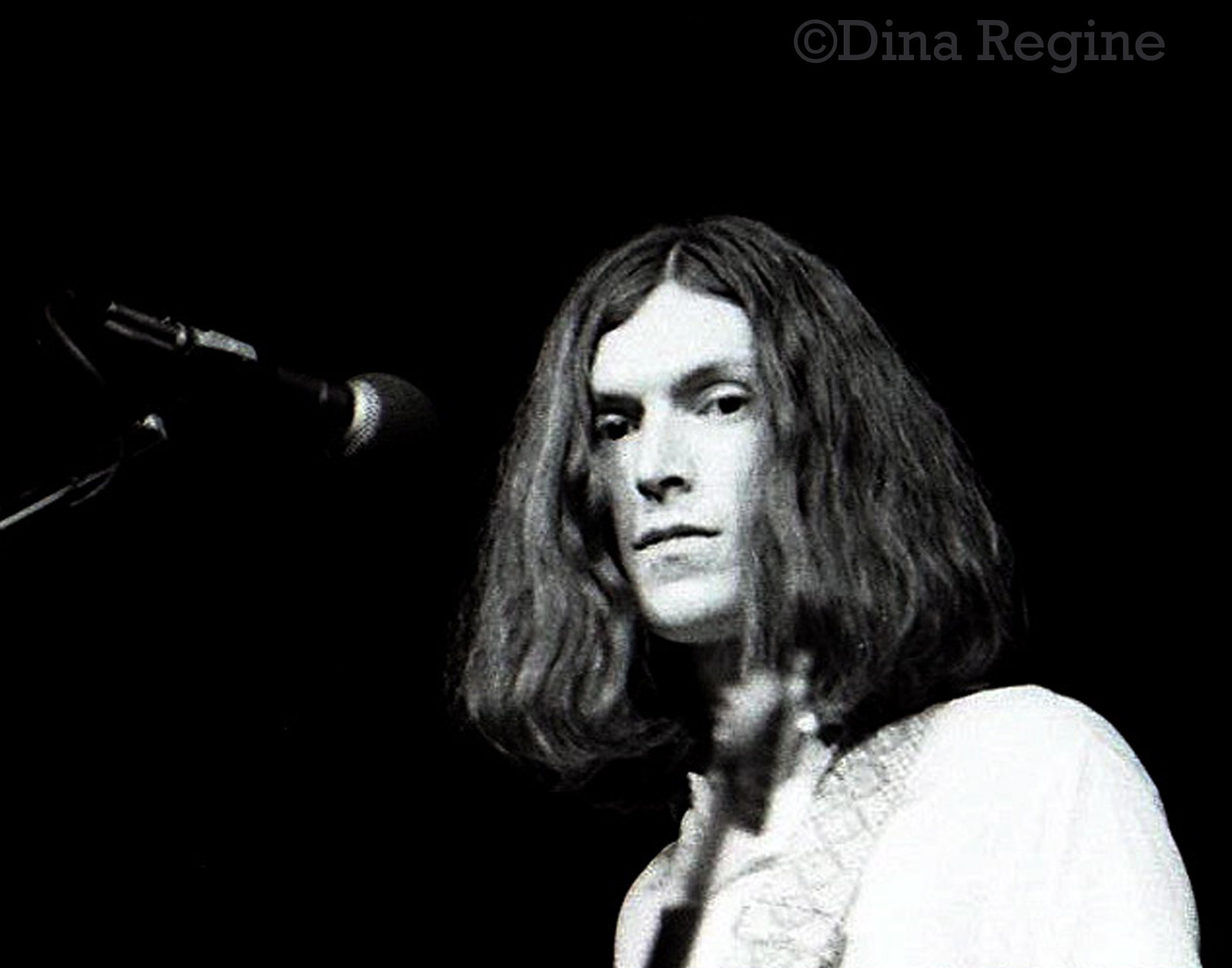This black and white photograph captures a moment of a musician, possibly a young Steve Winwood, performing on stage. The musician, dressed in a white shirt and wearing a decorated guitar strap over his left shoulder, is playing a guitar, with only the head and neck of the instrument visible due to the slight blurriness of the image. His long, thick, shoulder-length hair, characteristic of the 1960s hippie style, falls naturally around his face. He appears to be looking down towards the viewer with a somewhat indifferent expression. A black microphone with a silver tip extends towards him from the left side of the image. The background is entirely black, emphasizing the figure of the musician. In the top right corner, the photo is marked with gray text that reads "© Dinah Regine."